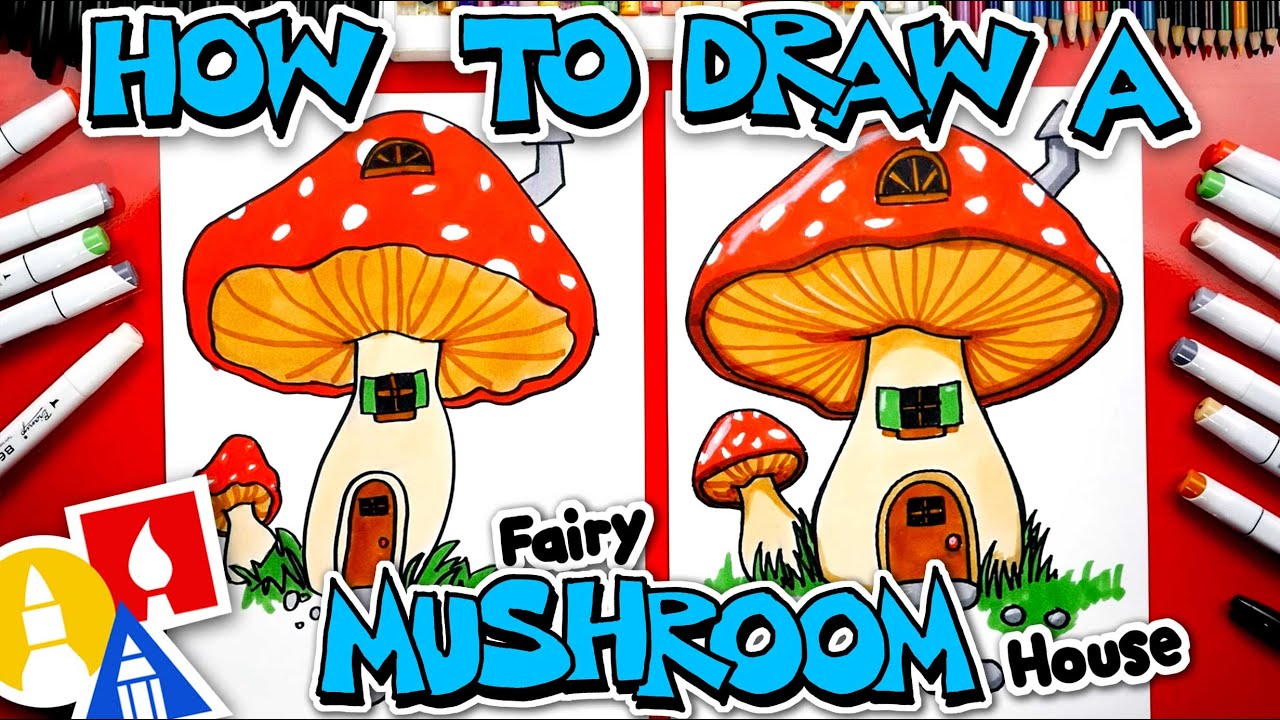The image is a rectangular illustration, wider than it is tall, showcasing side-by-side drawings of fairy mushroom houses on white papers placed on a red table. The top of the image features large blue block letters with black shadowing and a white border, stating "How to Draw a." Below it, in smaller text, it reads "fairy mushroom house." Both drawings depict nearly identical whimsical mushroom houses with red caps adorned with white polka dots, yellow underbellies, chimneys on top, brown doors on the mushroom stems, and windows above the doors. There is also grass and a smaller mushroom next to each house. At the bottom left corner of the image, three colorful icons are depicted: a blue triangle, a yellow circle with an art utensil motif, and a red square with a fire emblem. Additionally, colored markers are visible on either side of the papers and the tips of colored pencils are arranged along the top of the image.